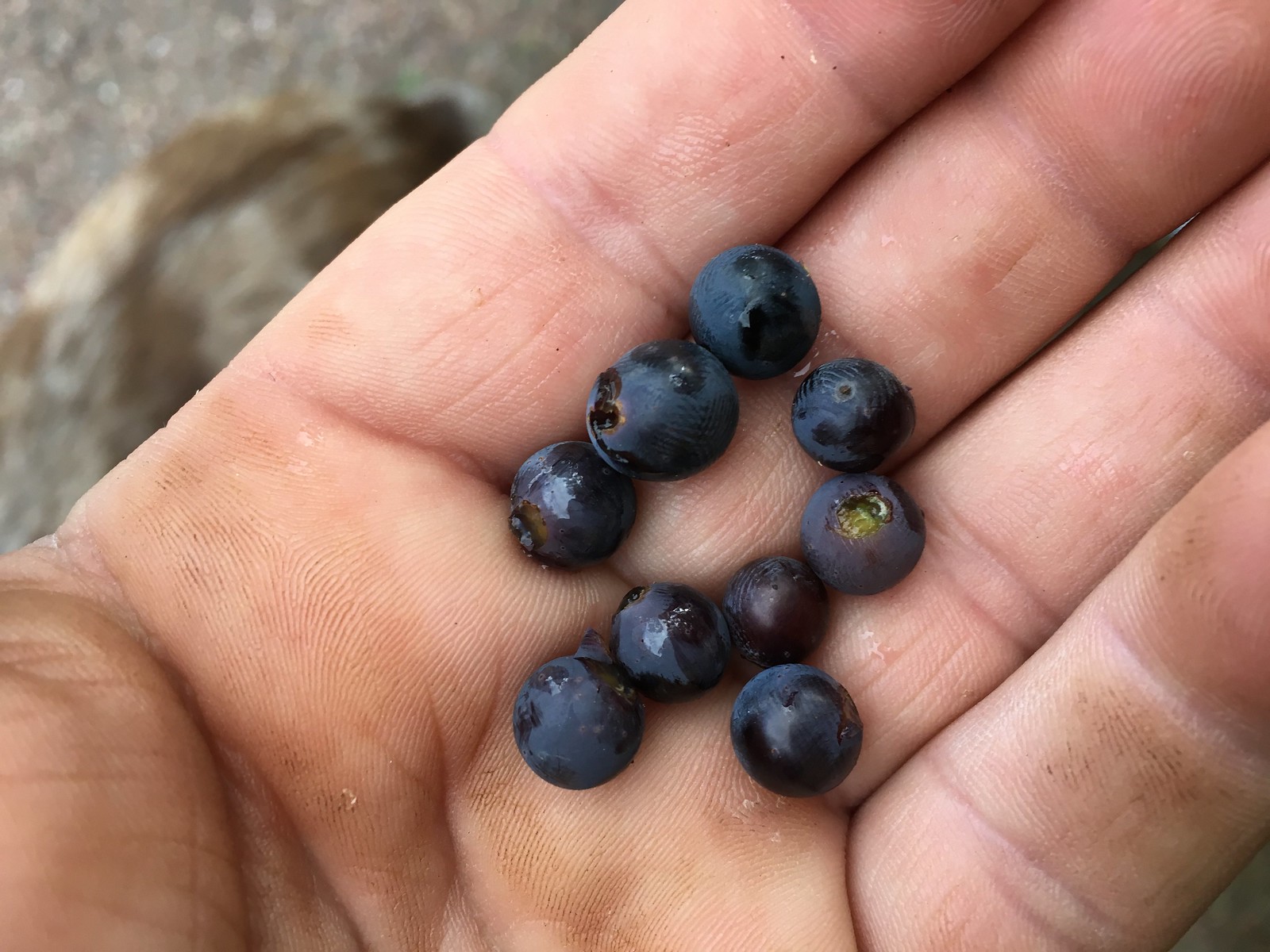This is a detailed, high-definition close-up photograph of a Caucasian male's left hand from the palm side, slightly slanted with the thumb not visible. The hand, which shows a bit of dirt around the pinky finger, is holding nine tiny, freshly picked blueberries. The blueberries have some water droplets on them and are mostly gathered near the middle finger, close to the part of the palm near the fingertips. The background, though out of focus, indicates an outdoor setting with what appears to be gravel or concrete and a part of a dog's body visible in the top-left corner. The hand occupies the majority of the image, leaving small sections of the brownish background visible in the bottom right and top left corners.